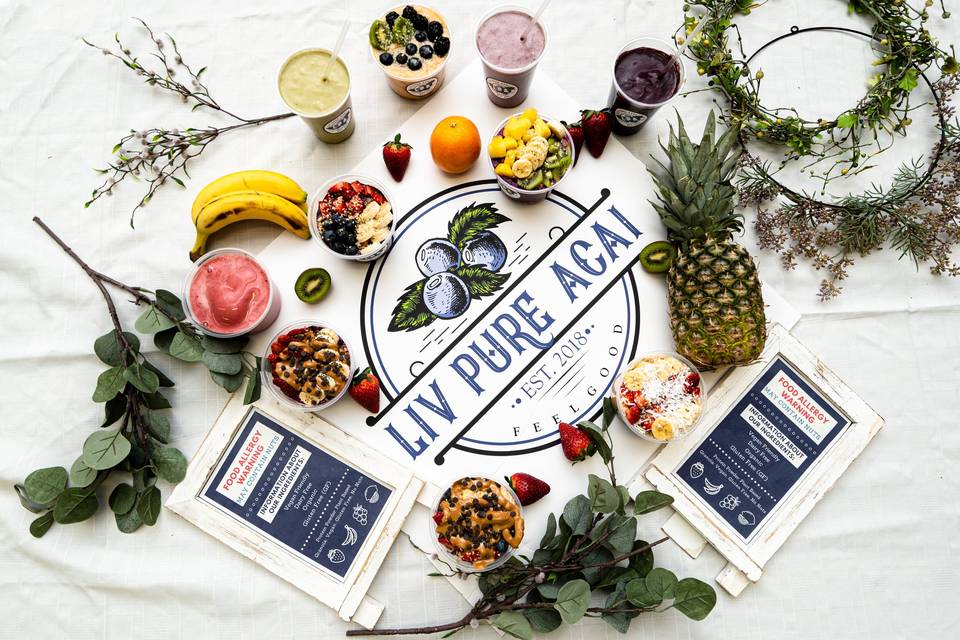This overhead photograph showcases an inviting advertisement for a health-focused food brand named "LIV Pure Acai," established in 2018. The backdrop is a pristine white tablecloth, providing a clean canvas that highlights a central logo featuring a blueberry and adorned with the brand's name in blue text. The logo also includes the inspiring motto "Feel Good." Surrounding the logo is an abundant spread of colorful fruits and smoothies, enhancing the theme of pure, wholesome eating.

The table is elegantly arranged with bowls of assorted fruits such as bananas, kiwis, strawberries, oranges, pineapples, papayas, and shredded coconut. Various vibrant smoothies, including green, lavender, and dark purple ones, are strategically placed to showcase the brand's refreshing offerings. In addition to the fresh ingredients, there are packages that likely contain the product's smoothie mixes, accentuated with labels highlighting key attributes such as allergy warnings, vegan-friendly, dairy-free, organic, and gluten-free information.

Festive elements like wreaths and branches are sprinkled around, enhancing the visual appeal and reinforcing the brand's commitment to natural, healthy living. The overall composition of the image effectively conveys a message of vitality and wellness, inviting viewers to "Feel Good" with LIV Pure Acai.